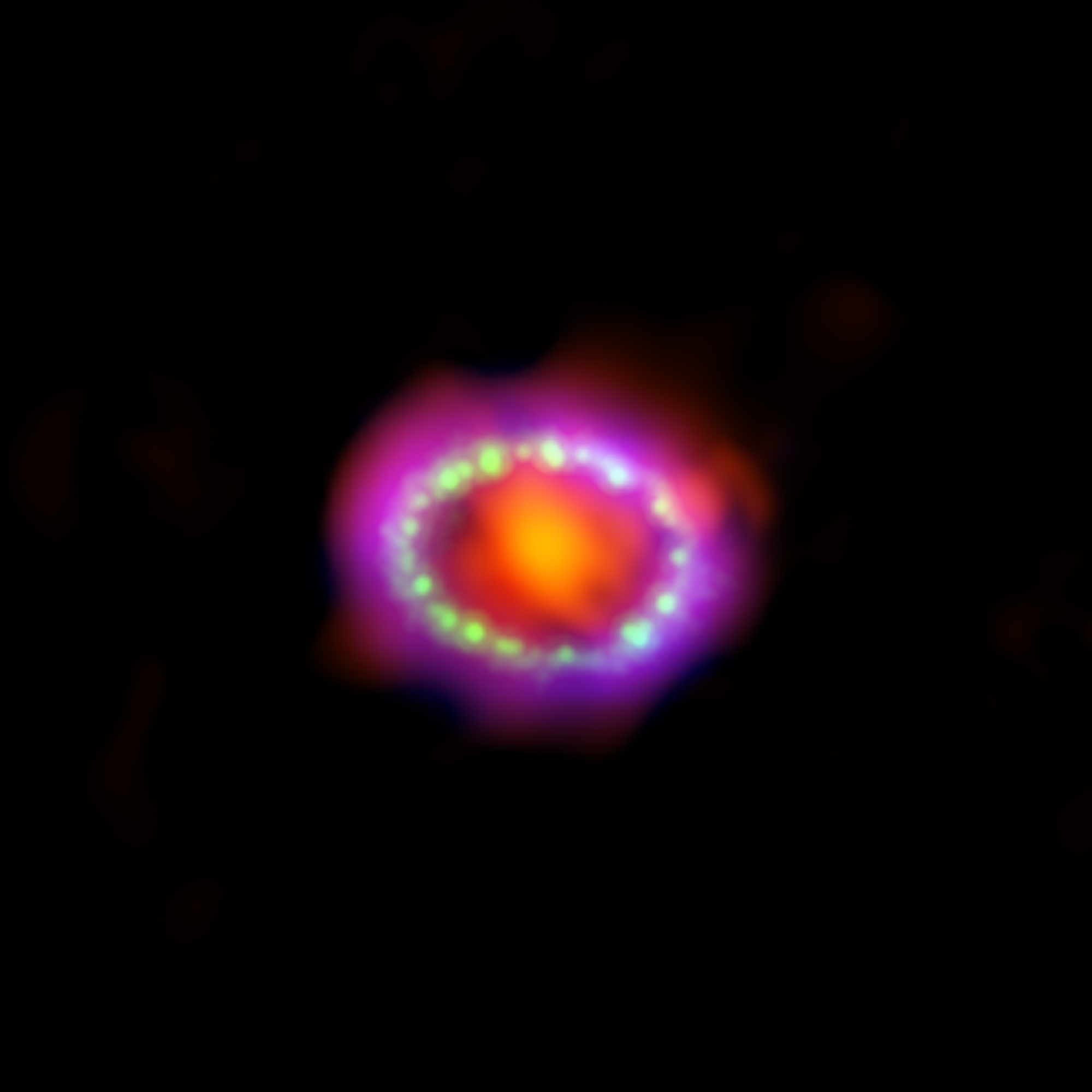The image depicts an enigmatic, unfocused light source or celestial body set against a completely dark, black background. The central feature is a cloudy, circular, hazy orb with a vibrant array of colors. The outermost ring exhibits a gradient of red and purple hues, creating a smoky texture around the edges. Inside this ring, there's a layer exhibiting a delicate pearl necklace-like pattern in green and white, reminiscent of stars or bright explosions in space. The innermost part of the image is dominated by a larger, bulbous area with fiery yellow and orange tones, giving it the appearance of the blazing sun or a burst of light. This combination of blurred colors and patterns makes the image resemble a telescopic view of a celestial phenomenon, such as a galaxy or a fractal design, though its exact nature remains ambiguous.